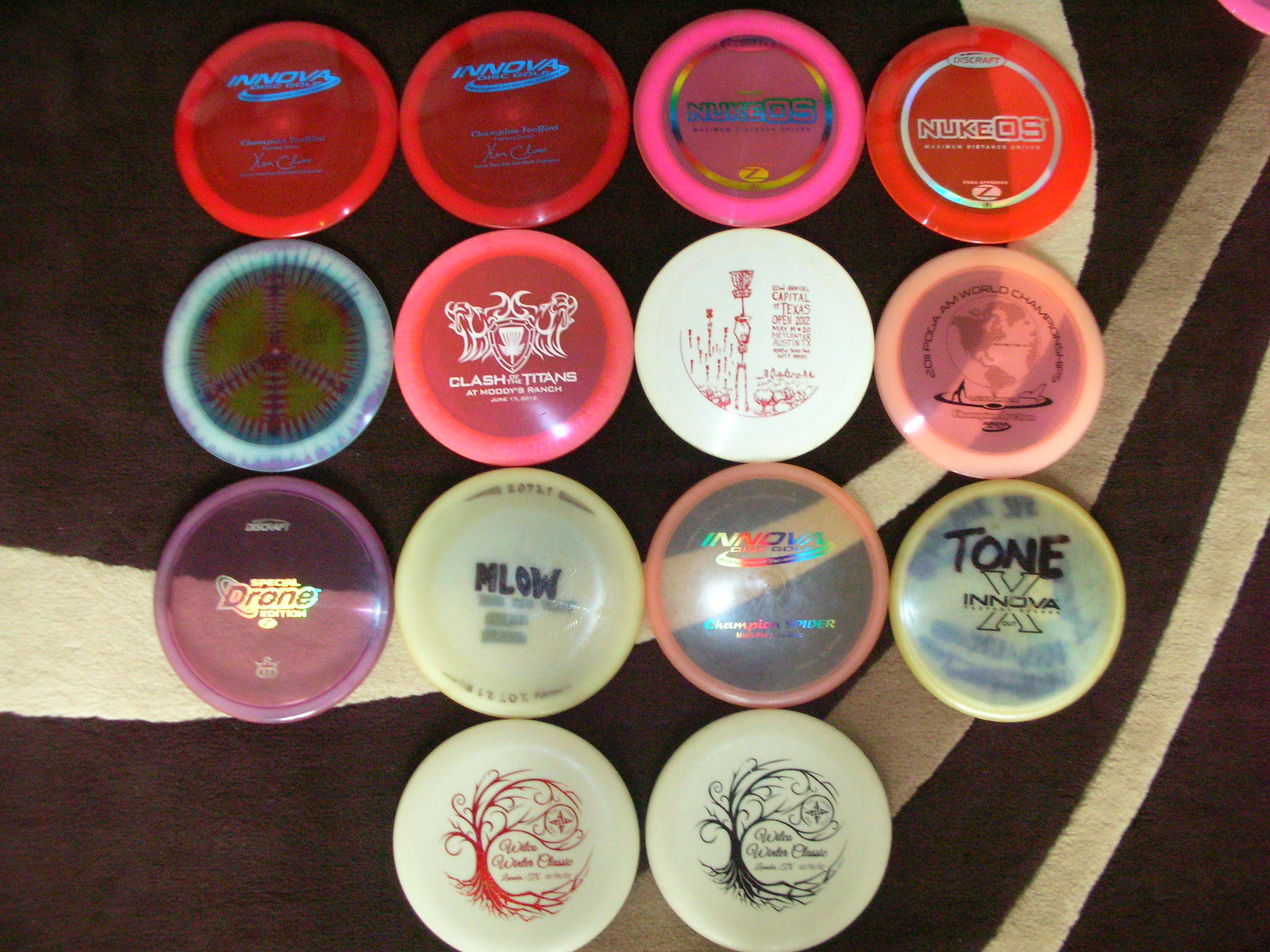This image features an array of small plastic discs, resembling pogs or poker chips, meticulously arranged on a black carpet with a thick white pattern. The discs are organized in three rows of four, with an additional two discs centered at the bottom. Each disc is distinctly colored and adorned with unique logos or text. Starting from the top left, the first disc is red with blue text reading "Innova." This is followed by another red disc with a silver outline and the words "Nuke OS" in silver. The next disc is pink with blue text and a rainbow outline, while the fourth in the first row is red with blue "Innova" text.

In the second row, a blue disc features a tie-dyed peace sign at its center. Next, a pink disc is inscribed with "Clash of Titans," and a white disc showcases red text, mentioning "The Capital of Texas Open 2002." The final disc in this row is a light pink one with a faint black globe and small black lettering surrounding it.

The third row introduces a light purple, transparent disc with the word "Drone" in silver text, followed by a whitish-yellow disc that appears to glow in the dark with "Enblow" written in black. Another clear light pink disc features "Innova" in shimmery rainbow letters, and the last disc in this row is white with "Tone" written in black marker, accompanied by another "Innova" logo.

Finally, the bottom row consists of two discs, one white and one black, both featuring a red tree.